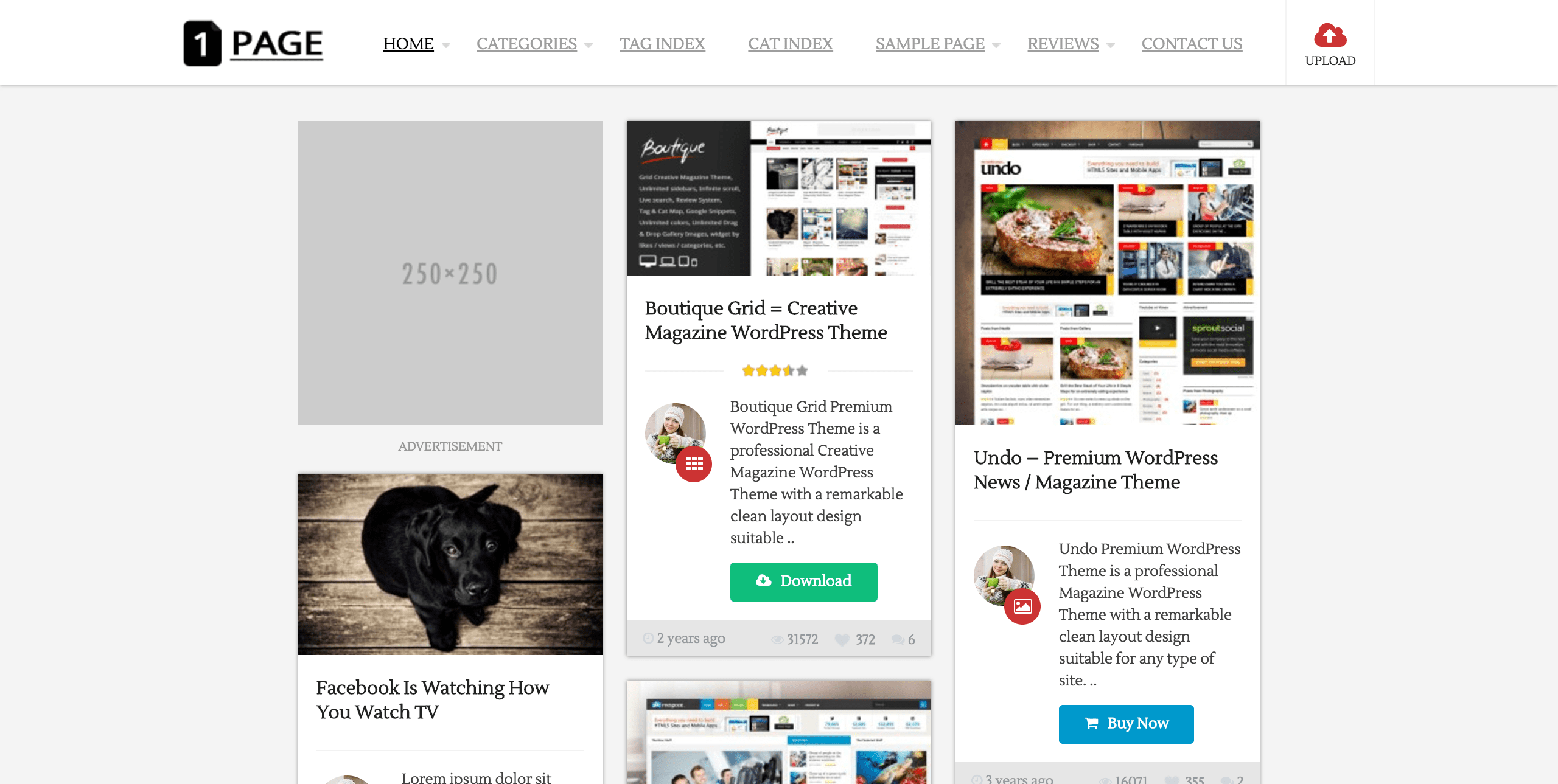**Caption:**

This image is a detailed screenshot of a WordPress template named "OnePage." In the upper left corner, there is a distinctive icon: a black rectangle with a dog-eared corner, featuring a white numeral "1" inside it. Next to this icon, the word "PAGE" is prominently displayed in uppercase letters, underlined in black.

Below this header, a comprehensive navigation menu is shown, which is set against a white background and underlined with a grey bar. The "HOME" button is selected and highlighted in black, while the rest of the menu options—"CATEGORIES," "TAG INDEX," "CAT INDEX," "SAMPLE PAGE," "REVIEWS," and "CONTACT US"—are grey and underlined. Each menu item is written in capital letters, ensuring a uniform appearance. Additionally, there's a red cloud icon with an upward-pointing arrow labeled “UPLOAD.”

In the upper left section of the main site, there is a placeholder for a 250 by 250 pixel advertisement. Below this advertisement space is an image of a dog standing on a wooden floor, looking up. Superimposed on this image is the text: "Facebook is watching how I watch your TV."

At the center of the layout, there's a panel titled "Boutique Grid Creative Magazine WordPress Theme," which displays another screenshot, creating a meta-screenshot effect. On the right panel, a separate section labeled "Undo" highlights a premium WordPress theme for news and magazines. This section includes rating indicators, some placeholder dummy text, and two essential action buttons: "Download" and "Buy Now."